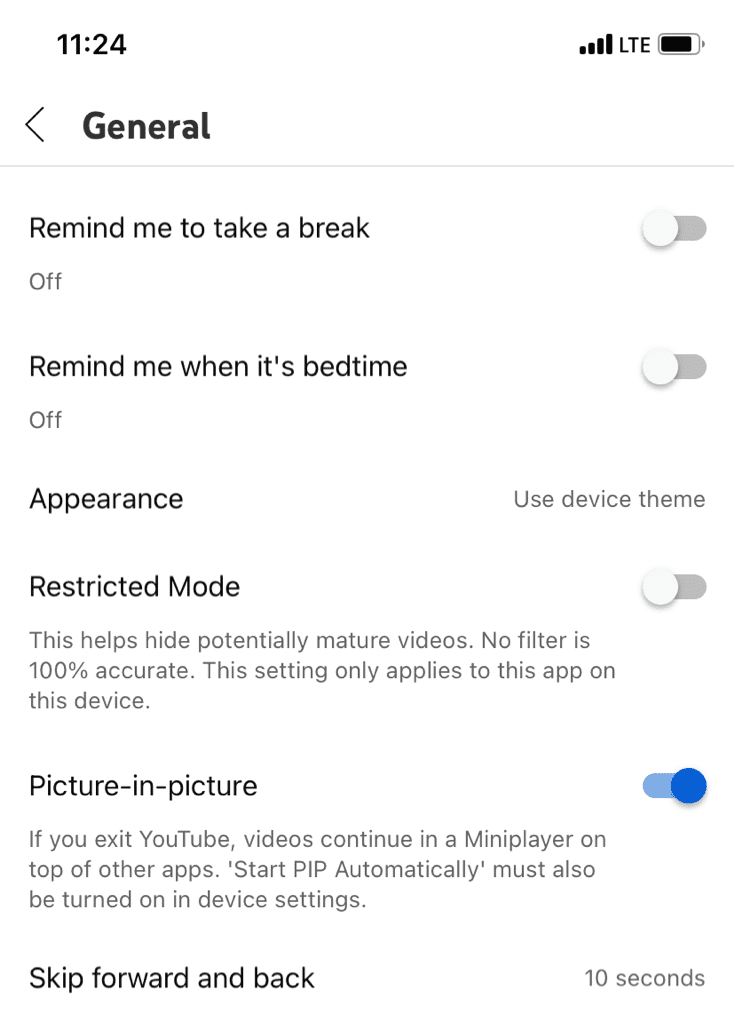**Caption:**

A screenshot of a phone displaying a settings menu under the "Websites" category. The time shown on the phone is 11:24, without specifying AM or PM. The phone is connected via LTE with no Wi-Fi, and the battery is approximately 80% charged. At the top of the screen, there's a "General" label with a backward arrow next to it, indicating navigation to a previous menu. Below this, various toggle options are visible:

1. "Remind me to take a break" - This option is turned off.
2. "Remind me when it's bedtime" - This option is also turned off.
3. "Appearance" - Set to "Use device theme."
4. "Restricted mode" - Described as a feature to help hide potentially mature videos, with a note that no filter is 100% accurate and it only applies to the app on this device. This setting is turned off.
5. "Picture-in-picture" (PIP) - Allows YouTube videos to continue playing in a mini player while using other apps. It notes that PIP must be enabled in the device settings for it to start automatically. This setting is turned on.
6. "Skip forward and back 10 seconds" - This option is also enabled.

All toggles except for "Picture-in-picture" and "Skip forward and back 10 seconds" are set to gray, indicating they are off, while the enabled options are highlighted in blue.